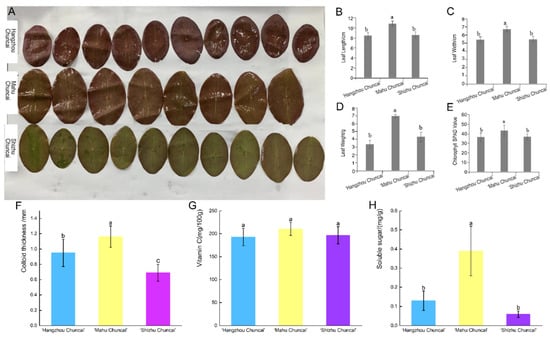The image displays an intricate arrangement, featuring a background with brown and dark green colored ovals that could be mistaken for leaf-like shapes or possibly rocks, giving it a textured appearance. Overlaying this background are numerous bar charts arranged in three rows and labeled B, C, D, E at the top, and F, G, H at the bottom. Each chart showcases colored bars in sequences of turquoise blue, yellow, magenta, and purple, with some repetition of these colors. The general background of the image is primarily white, although some elements and the middle part of the bars are softly tinged with yellow. The horizontal and vertical axes contain text that is too blurry to decipher clearly, hinting at various types of information, possibly in a different language. The overall scene suggests a detailed and visually complex statistical or analytical presentation, despite the difficulty in reading the finer details.